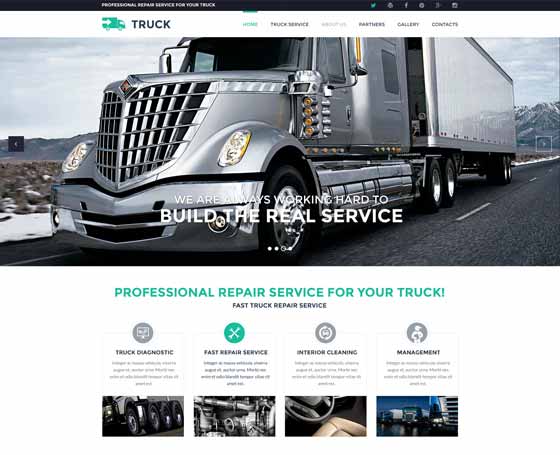On the website, a prominent image of a gray semi-truck dominates the center, appearing to move slightly leftward and towards the viewer. This semi-truck is hauling a storage container and features five visible wheels on its left side, with the right-side wheels not shown. At the top of the webpage, a thin black bar contains a series of icons and white text, though they are not clearly visible due to low image quality. The site’s background above the truck image is white. In the top left corner, the word "Truck" is displayed in black text, while the top right corner features navigation buttons labeled "Home," "Truck Service," "Partners," "Gallery," and "Contacts."

Across the truck image, the phrase "We are always working hard to build the real service" is displayed in bold white text. Beneath this image, the background shifts to white with green text proclaiming "Professional repair service for your truck." Below this, a black subtext reads, "Fast truck repair service." Further down the page, there are four sections in columns detailing varied services: "Truck Diagnostics," "Fast Repair Service," "Interior Cleaning," and "Management." Each service is accompanied by a brief four-line description in small gray text, and relevant images are displayed underneath each service description.